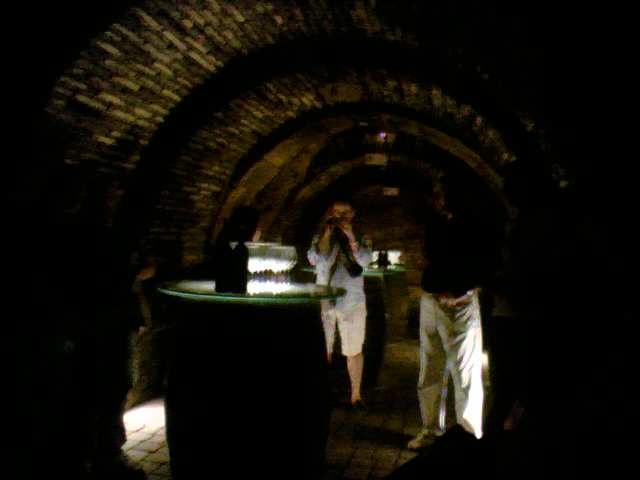The image is a blurry, rectangular photograph of a dark, underground tunnel-like room constructed of black, yellow, and brown bricks. The arched ceiling of the tunnel is supported by possibly wooden beams at intervals. The room is very long, with a series of round, bar-height tables featuring glass tops that are illuminated from underneath. These tables display several wine glasses and possibly wine bottles. In the image, there are two people: a woman in a white outfit that includes a robe, and a man in a dark top with khaki pants. The woman appears to be taking a photograph, raising a dark object to her face. Light streams in from the top and sides of the tunnel, adding a faint blue glow to the scene. The overall dark and blurry quality of the photo makes it challenging to discern finer details, but the setting suggests an intimate, possibly subterranean event space.